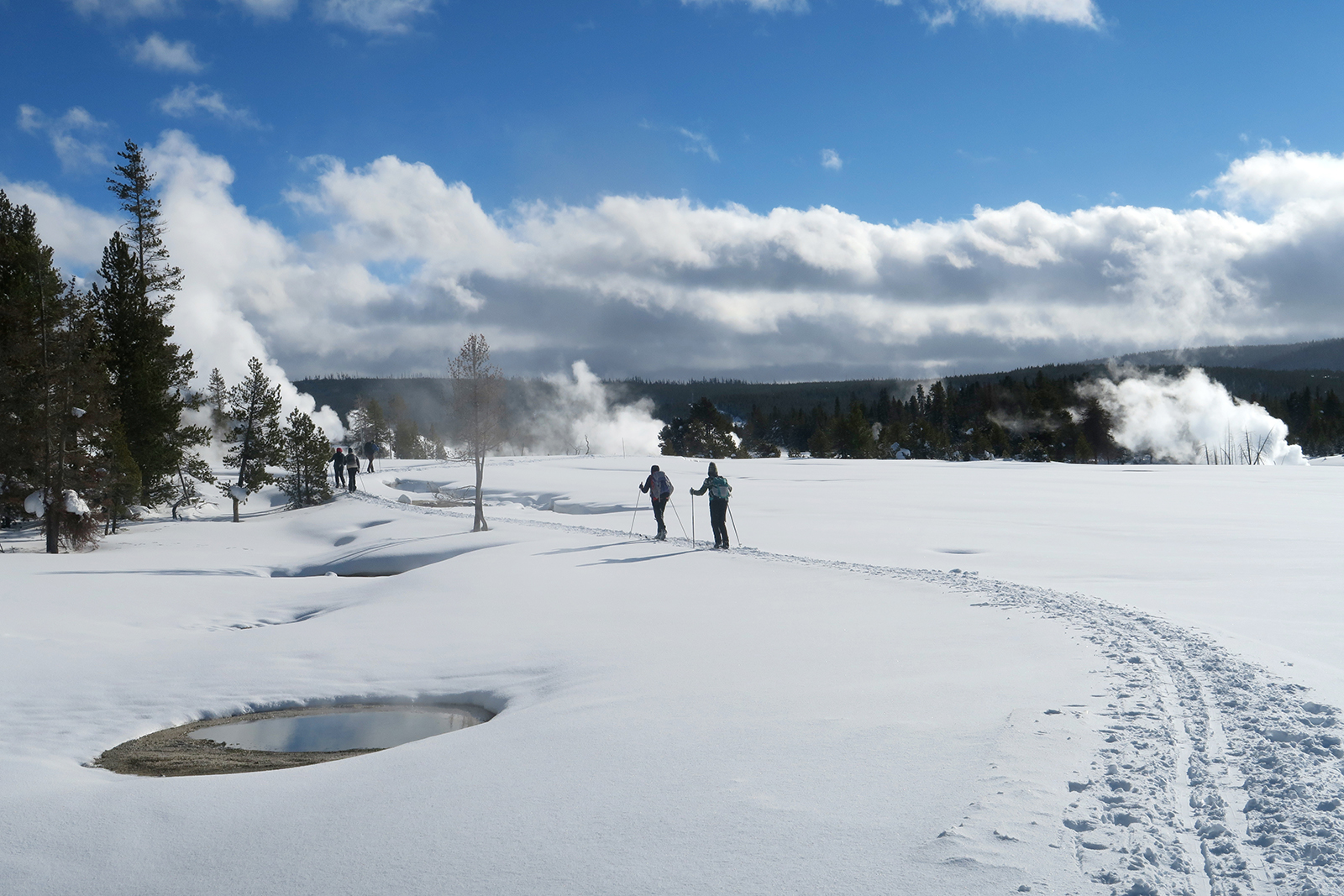The image captures a bright, snowy landscape under a partly clear, blue sky with fluffy clouds scattered. In the foreground, two people are seen navigating the flat terrain with ski poles, following a path marked by tire tracks and footprints carved out in the fresh snow. Ahead of them, at least three more individuals are scattered along the same path, also using ski poles. To the left side of the image, a notable feature is a small puddle of exposed water, possibly a hot spring, as steam can be seen rising from its surface. This puddle, surrounded by untouched white snow, reveals some greenery around it. The background of the image features a horizon lined with dark pine trees, with distant hills or mountains adding depth to the scenery. The overall scene is bright and clean, with the untouched snow contrasting against the dark, tree-lined horizon.